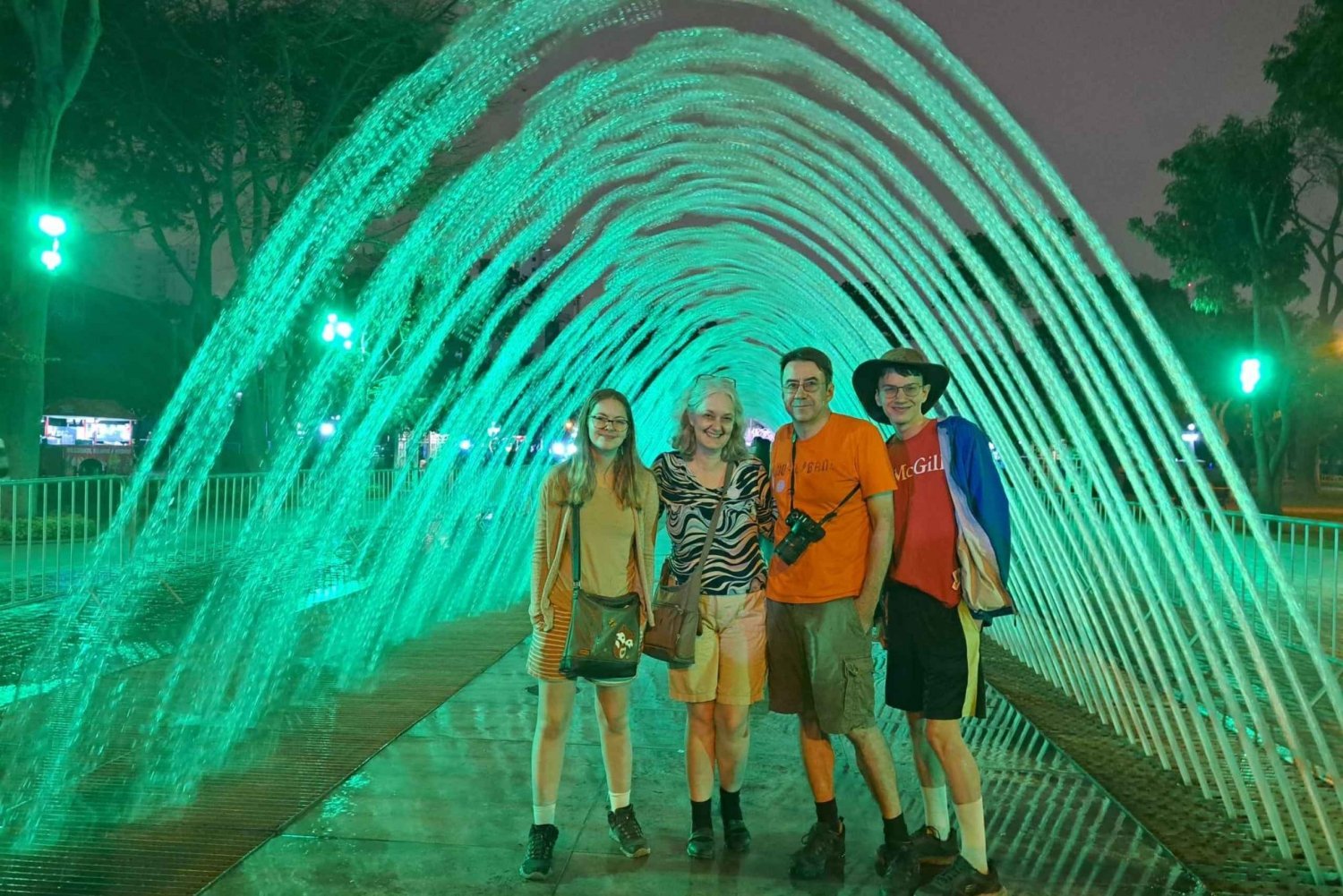A family of four is posing happily under a mesmerizing water archway installation at night, with the sky and trees visible in the background. The tunnel is formed by numerous water jets—possibly 50 to 100—shooting up from the ground and creating a protective arc overhead, which ensures that the family remains dry. The water jets are beautifully illuminated with a bright aqua and green glow, adding a magical effect to the scene.

In detail, the father stands to the left, wearing an orange t-shirt, shorts, and a camera slung around his neck. Next to him is the mother, dressed in a black and white patterned top, yellow shorts, and shoes, holding a purse. The son, standing to the right of the father, is wearing a red McGill t-shirt, a blue jacket, shorts, and a cowboy-like hat. The daughter stands to the right of the mother in a cheerful yellow top, a skirt with yellow and red horizontal lines, sneakers, and a purse. The family looks in their 50s for the parents and early teens for the kids, and all are smiling, clearly enjoying their time together in this enchanting setting.